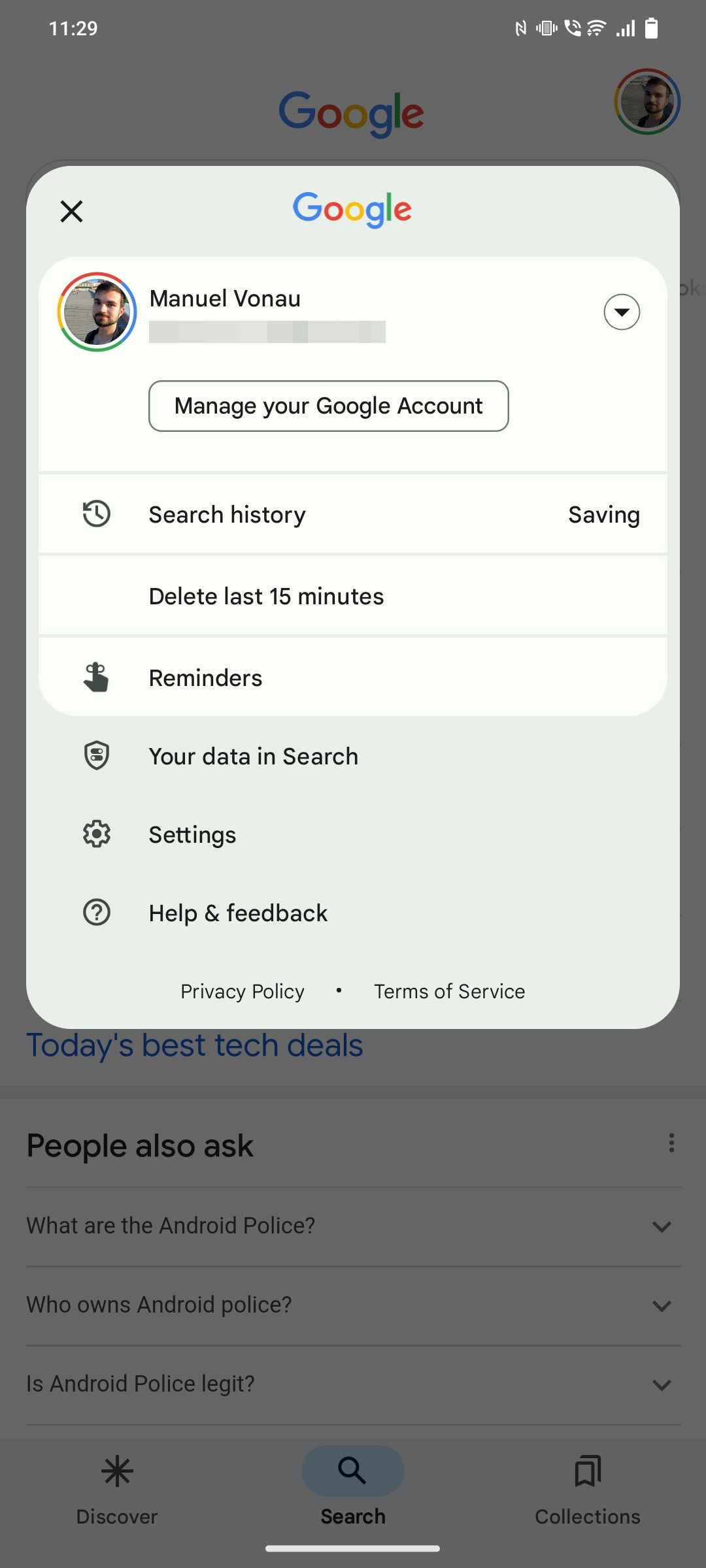A detailed screenshot from a smartphone, captured at 11:29 AM, illustrating a Google profile page for "Manuel Von Au, Vonov." The top left corner displays the time. The profile picture, set within a circle bordered by Google's iconic colors (blue, red, yellow, and green), features an image of a man. The screen prominently shows the "Manage your Google Account" menu, which includes options such as: "Search history," "Delete the last 15 minutes," "Reminders," "Your data in Search," "Settings," "Help," and "Feedback." The background of the image is slightly darker, highlighting the active overlay of the Google account management interface. Along the bottom of the screen are three tabs: "Discover" on the left, "Search" in the center, and "Collections" on the right.